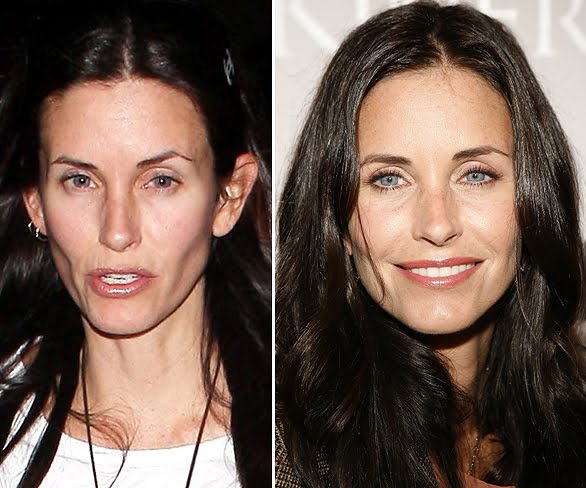The image presents a split-screen comparison of actress Courtney Cox, with two photographs placed side by side, likely intended to highlight a significant transformation in her appearance over time. The photograph on the right showcases a more polished, vibrant version of Courtney, with her fuller, elegantly styled hair cascading around her shoulders. Her bright blue eyes are strikingly prominent, complemented by a broader, more radiant smile and a well-applied professional makeup job, exuding confidence and grace.

In stark contrast, the photograph on the left depicts her with a less glamorous look, presenting as an older, fatigued version with stringy, unkempt hair and minimal to no makeup, contributing to a more anxious and wiry expression. Her lips are slightly parted as if about to speak, and her overall appearance is more frail and unhealthy looking.

Together, these images emphasize the stark differences in her appearance, possibly suggesting a dramatic makeover or contrasting moments in her life, giving insight into the impacts of makeup, styling, and possibly even lifestyle or health changes.